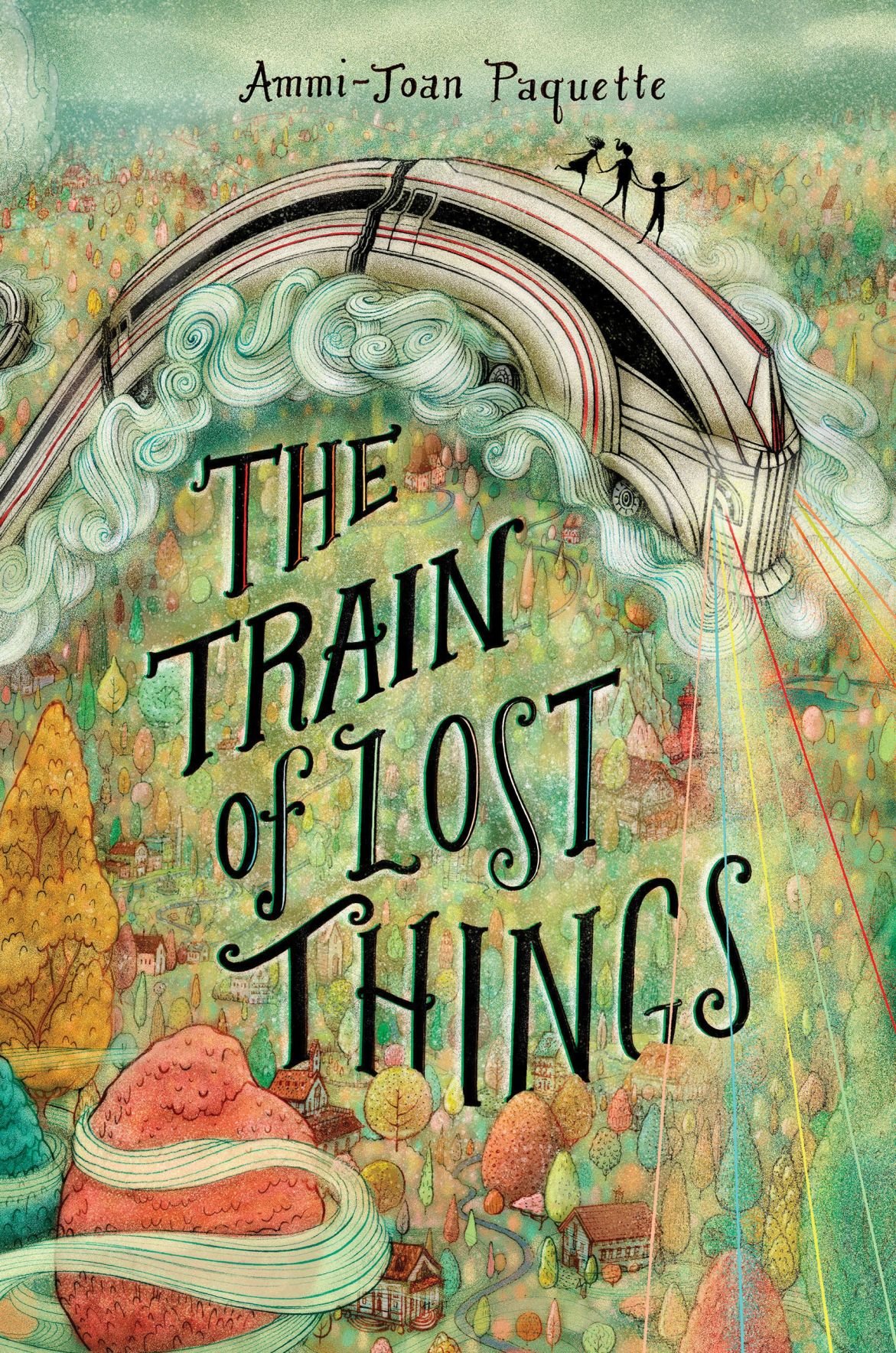The image is likely the detailed, whimsical cover of a book by Ami-Joan Paquette titled "The Train of Lost Things." Dominating the scene is a magical train, curving from the left side of the cover to the right. The train, illustrated in white and black with red stripes, appears to be flying through a green, cloud-like landscape, leaving behind plumes of clouds or dust. On top of the train, three shadowy figures are holding hands, with the leftmost figure raising one leg in the air, adding to the sense of wonder.

The environment is vividly colorful, featuring diverse trees in shades of red, orange, green, and blue scattered across a sprawling green landscape. Among the trees are houses and winding rivers and paths. The train is emitting multicolored rays of light—red, green, yellow, blue, and pink—from its front, enhancing the magical atmosphere. The author’s name, Ami-Joan Paquette, is printed in black text at the top, while the book’s title, "The Train of Lost Things," is prominently displayed at the bottom.